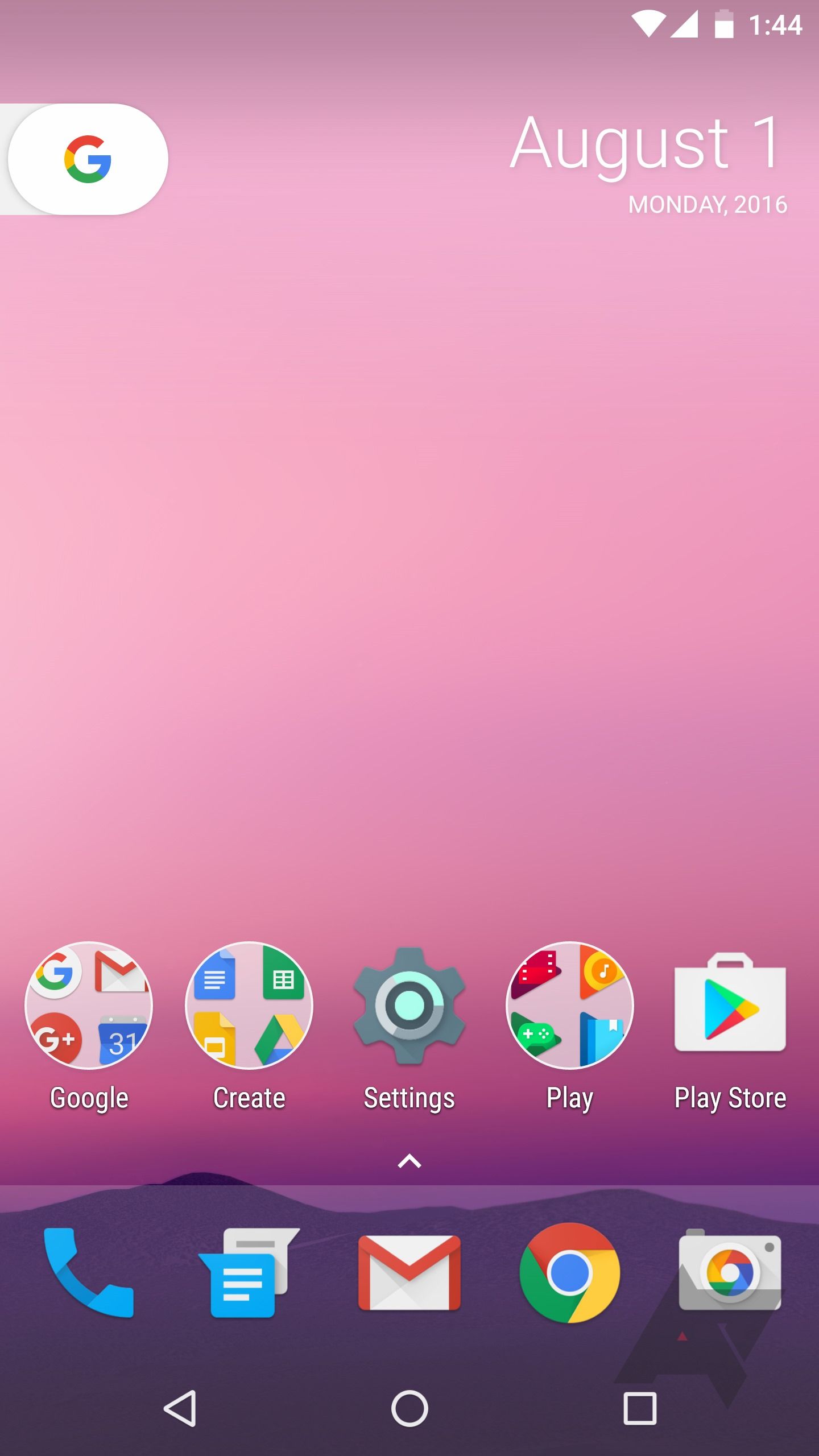The image depicts a phone screen wallpaper featuring a stunning ombre color gradient. The background transitions smoothly from a very light pink at the top to progressively darker shades of pink, culminating in a rich magenta, and finally blending into a foggy purple hue at the bottom. 

In the top right-hand corner, white icons for Wi-Fi and signal strength are displayed, along with a battery icon showing a charge around 70%. The time, indicated in white digits, reads 1:44. A Google search bar sits at the top of the screen with the iconic 'G' logo colorfully transitioning from red and yellow to green and blue.

To the right of the search bar, the date is displayed as 'August 1', while on the left, it states 'Monday, October 2016'. 

At the bottom of the screen, there are two rows of app icons. The first row includes labeled icons for 'Google', 'Create', 'Settings', 'Play', and 'Play Store'. The second row consists of unnamed icons including a blue phone icon, two text message icons (one blue and one grayish white), a white envelope with a red 'M' for Gmail, the Google Chrome icon with red, yellow, green, and blue colors, and the Google Photos icon, represented by a grayish white camera with a colorful circle.